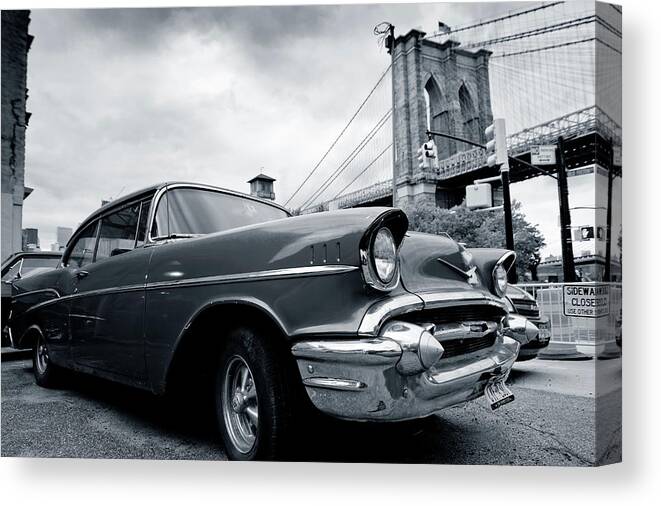This is a detailed black and white photograph of a vintage vehicle, likely from the 1950s or 1960s, taken from a low perspective looking up. The vehicle, a darker color with a chrome bumper and circular headlights, is a two-door model parked underneath a large bridge with two arches made of blocks, situated on the right-hand side. Adjacent to the vehicle, there is a sign that reads "SIDEWALK CLOSED" in black lettering on a white background, likely accompanied by smaller, blurry text that suggests "use other." Behind the car, a fence and a "SIDEWALK CLOSED" sign can be seen along with a large bush. On the left side of the image, a corner of a building is partially visible and below the bridge, stop lights and a crosswalk are present. The sky above is cloudy, adding to the overall moody ambiance of the photograph.